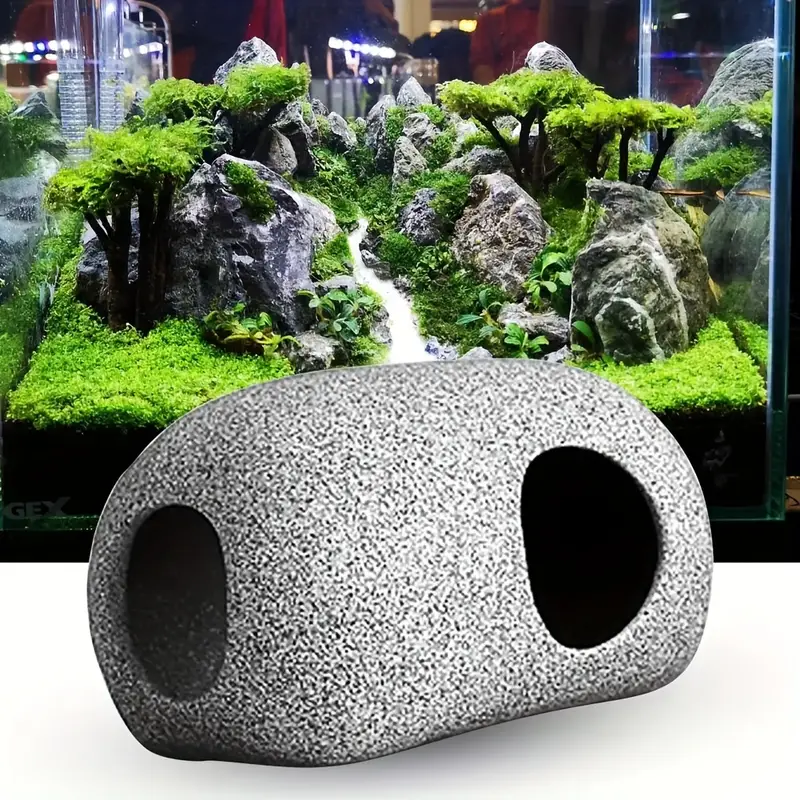The image depicts a miniature terrarium that intricately resembles a natural landscape. Dominating the foreground is a gray, stone-like object shaped like a mask, with two large, dark oval holes where the eyes would be. This digitally edited element has a textured appearance with white and black grains. The background features a lush, green environment enclosed in glass, containing various small trees and bushes atop rocky terrain. A stream or tiny waterfall runs through this miniature garden, flanked by multiple rocks of different sizes. The overall composition blends the stone mask and the terrarium, presenting a juxtaposition between the artificial and the natural elements within a digitally manipulated scene.